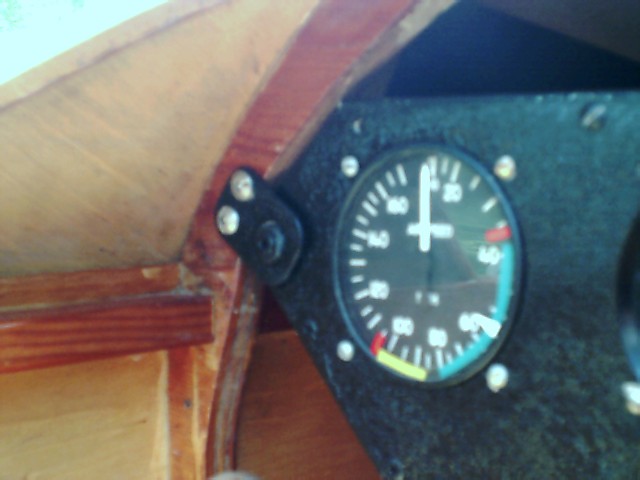The image showcases what appears to be a section of the cockpit, potentially from a small airplane or vintage car. The focal point is a black-rimmed dial mounted on a black plate, held in place by four silver screws. This dial, which features numeric markings and a needle, is securely fastened to a wooden frame, integral to the cockpit structure. The surrounding material looks to be either fiberglass or cloth, adding to the vintage aesthetic. On the right edge of the image, there's a partial view of another dial, but its details are obscured. A silver screw is also visible, contributing to the attachment of the dial to the dashboard. Additionally, a sliver of blue sky peeks through the upper left corner, hinting at the cockpit being of a small aircraft.